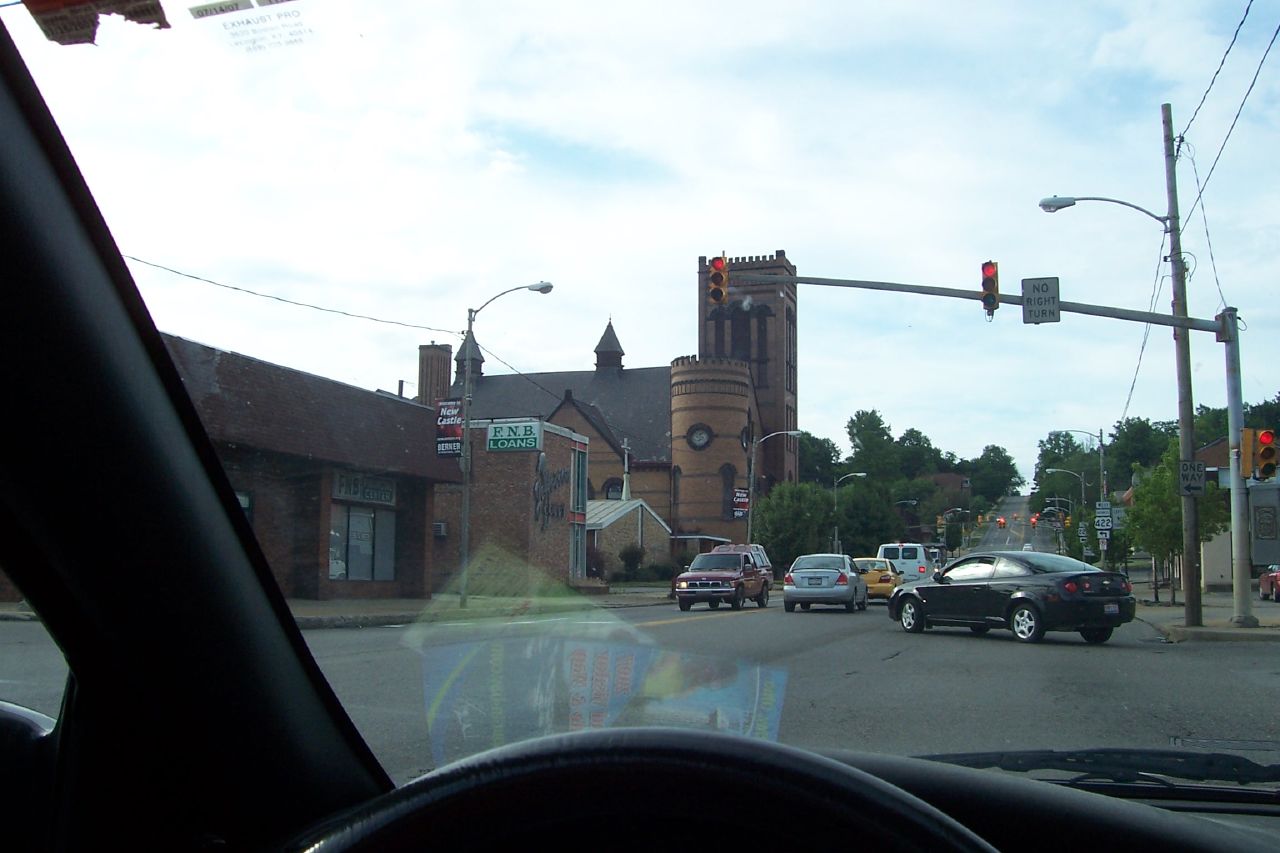The image captures the view from inside a dark gray or black car, looking out through the windshield over the driver’s side. In the foreground, the top of the steering wheel and the left door frame are visible, along with a subtle reflection from the dashboard that includes two brochures, one predominantly blue and another yellow. The windshield also displays a black wiper blade. Outside, the car is stopped at a red light with a visible "no right turns" sign. The street ahead is a busy, two-way road lined with trees and several buildings on both sides, including a prominently featured large church on the right with distinctive architecture: a tall front spire topped with a cross and a rounded, castle-like column. The building to the left displays a sign for "FNB Loans." There are multiple cars on the road: a black car, a silver sedan, a white sedan, and a white van all headed in the same direction as the car taking the photo, while a red pickup truck travels in the opposite direction. Additional elements include streetlights, telephone poles with wiring, and the clear daytime sky with white clouds against a light blue backdrop.